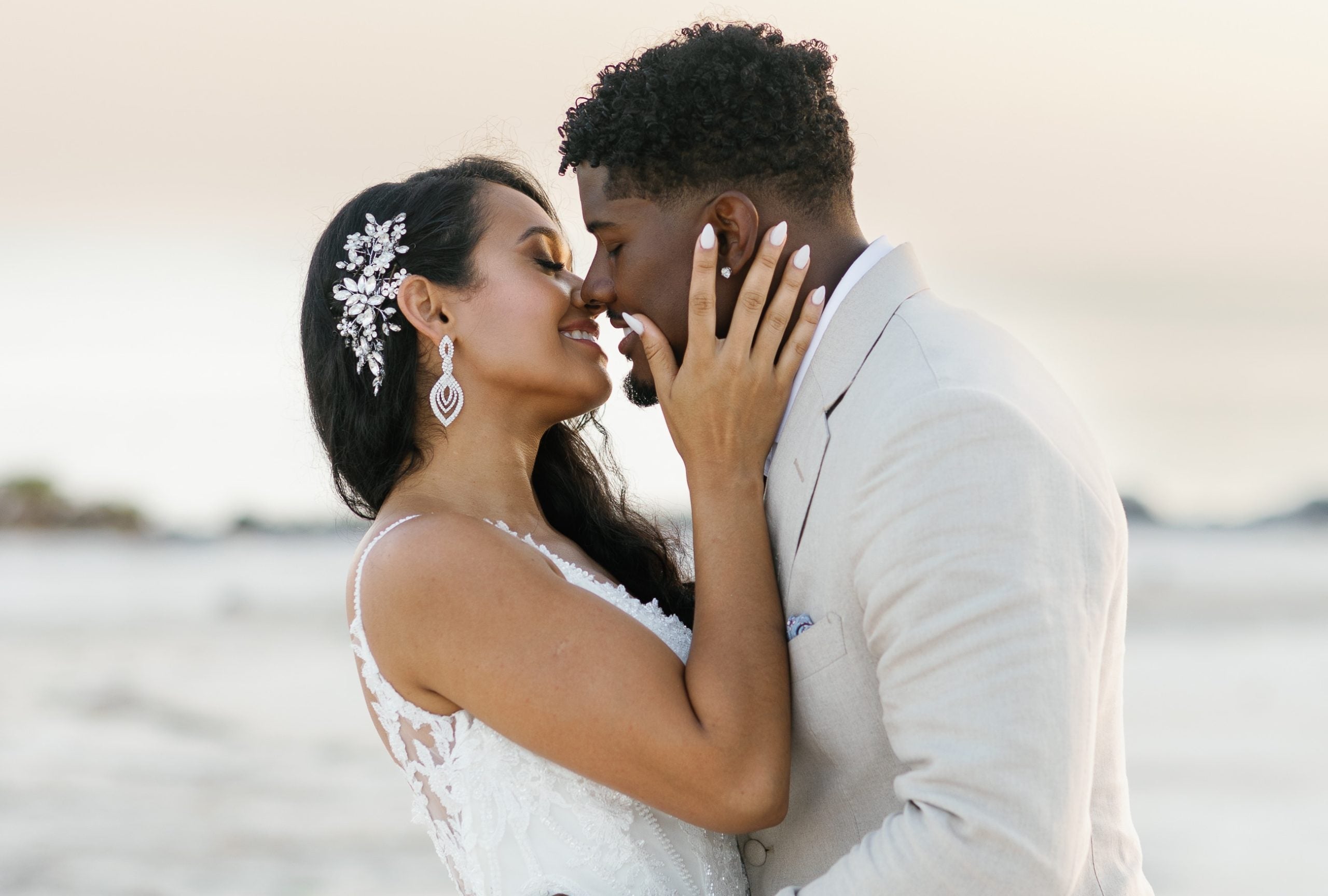In this image, a couple is captured in a tender moment by the water at sunset, exuding love and happiness. The young black man, on the right, is leaning in to kiss the woman with a radiant smile on his face. He wears a white and off-white suit with a light blue handkerchief in his breast pocket, and a studded diamond earring in his ear. His short curly black hair complements his elegant attire. The woman, positioned on the left, has long dark hair adorned with white flowers and rhinestones, enhancing her glowing appearance. She wears a white sleeveless dress, likely a wedding dress, along with large white earrings and white manicured fingernails. She lovingly holds his face in her hand while he wraps his hands around her waist, both smiling joyfully. The background showcases a beautiful, blurred depiction of water under the soft light of the setting sun.